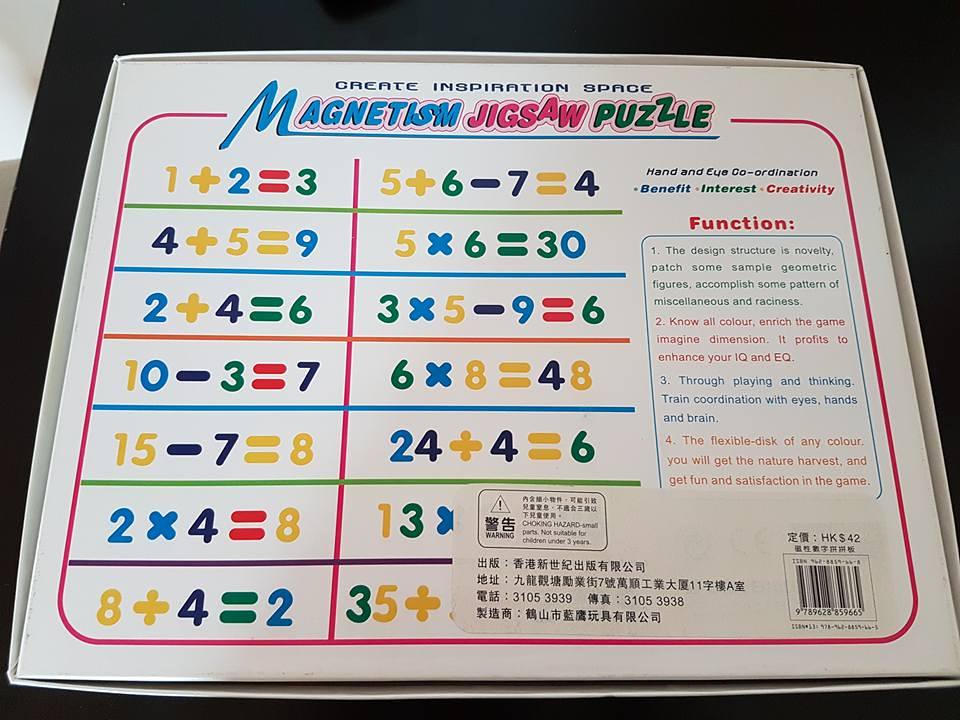The image depicts the bottom side of a game box against a black background, possibly on a table. The box is predominantly white and features colorful text in yellow, red, green, blue, black, and purple. At the top, it prominently reads "Create Inspiration Space, Magnetism Jigsaw Puzzle," followed by phrases such as "Hand and Eye Coordination, Benefit, Interest, Creativity." Central to the box's design is a chart displaying a sequence of math problems, ranging from simple equations like "1+2=3" to more complex ones like "3×5-9=6." These problems are presented in two columns with seven rows, each number and symbol uniquely colored. On the right-hand side are instructional and descriptive texts emphasizing the game's educational benefits and creative design, detailing activities like pattern completion and color recognition to enhance cognitive skills. At the bottom right corner, there is a price sticker in an Asian language, likely indicating a price of HK$42, which partly obscures some of the English text.